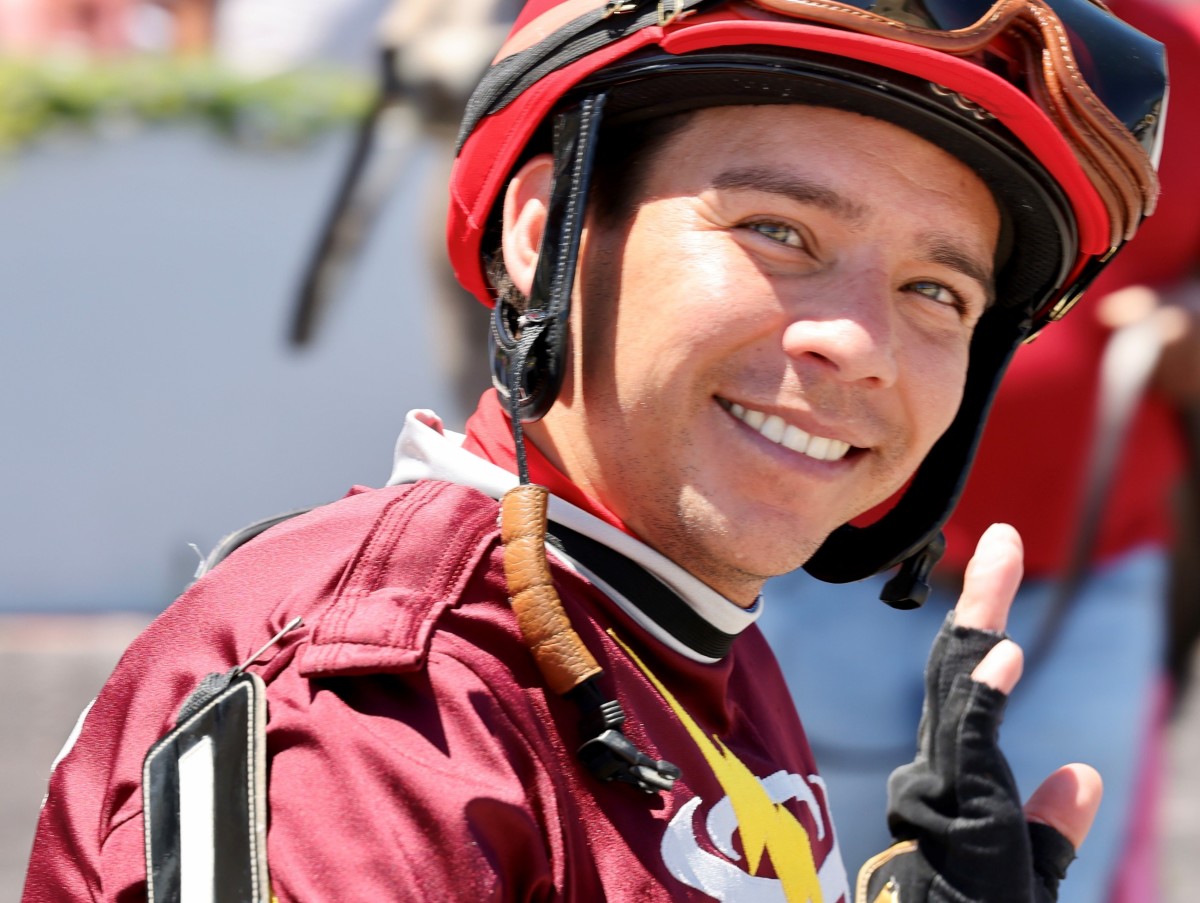This close-up image features a young Caucasian male, likely in his early 30s, who is smiling and waving at the camera. He has a slightly tanned complexion with a five o'clock shadow. He is dressed in traditional horse jockey attire: a red jockey helmet with mounted brown leather goggles placed above his eyes, black gloves with exposed fingers, and a maroon jockey jacket featuring shoulder flaps and a white graphic on the front. The man is the primary focus of the image, and though there appears to be someone standing behind him, along with a wall or gate, these details are blurred and not easily discernible.